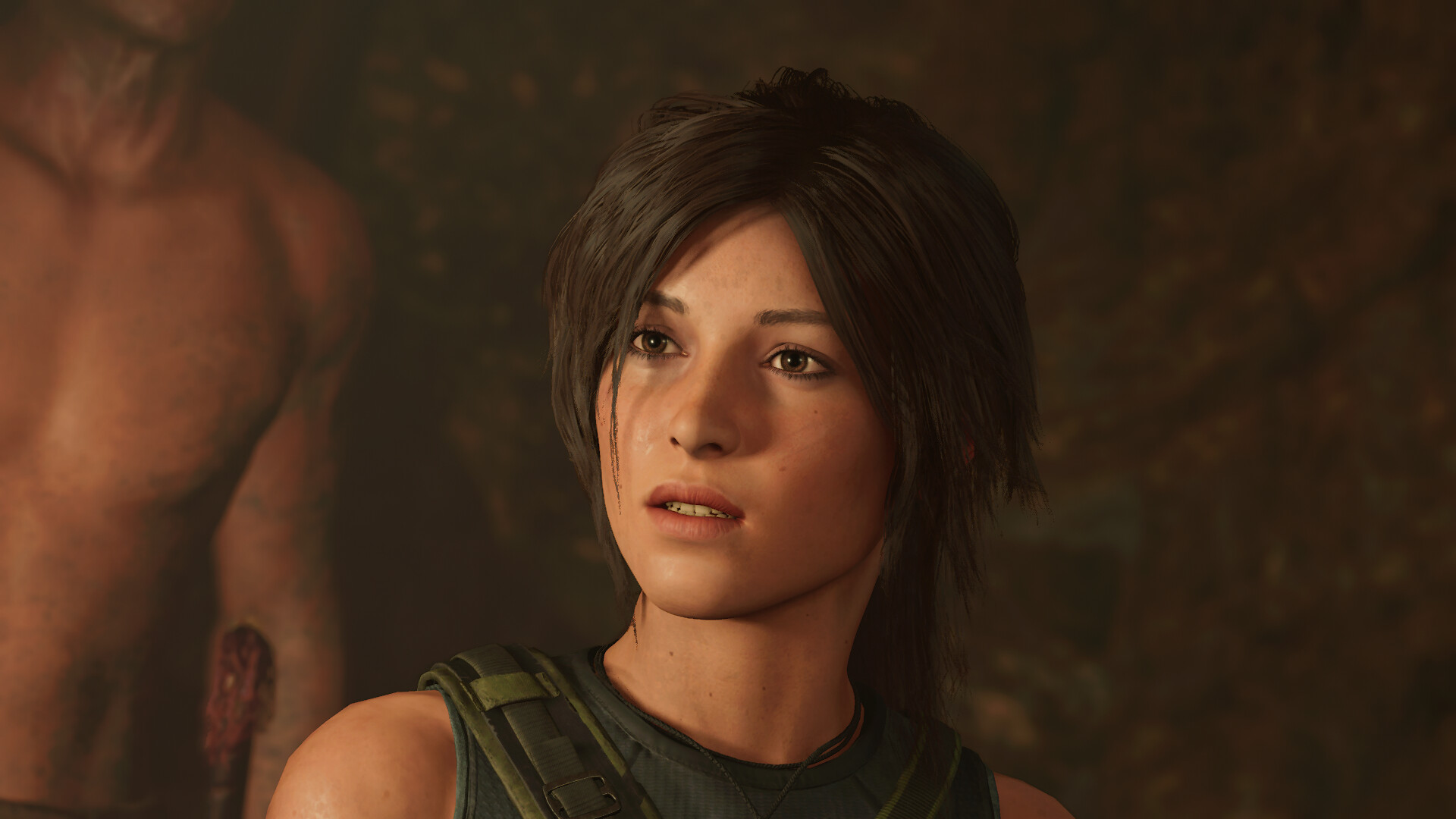The image is a high-quality screenshot from a recent video game, depicting the main character from the Tomb Raider series. The scene is horizontally rectangular, approximately twice as wide as it is tall. The central focus is the head and shoulders of a young woman, likely in her 20s. She has long, dark brown hair styled in a ponytail behind her neck, with a middle part and a wisp falling over one eye. Her facial expression is blank, and she gazes slightly to the right.

She is dressed in a forest green sleeveless top, possibly a military vest, with a strap from a shoulder bag visible over her right shoulder. Her skin is tanned, possibly with a few freckles. Her eyes are brown, and her overall appearance is distinct within the framed shot.

In the background, predominantly on the left side, is a shirtless muscular man, positioned very close to the woman as if creeping up on her. Although his head is out of frame, the visible parts of his left shoulder, chest, and arm suggest a powerful build. He appears to be holding an unseen object, as a wooden handle protrudes from his left arm past the elbow. The backdrop is a mottled dark brown, contributing to the dramatic and intense atmosphere of the scene.